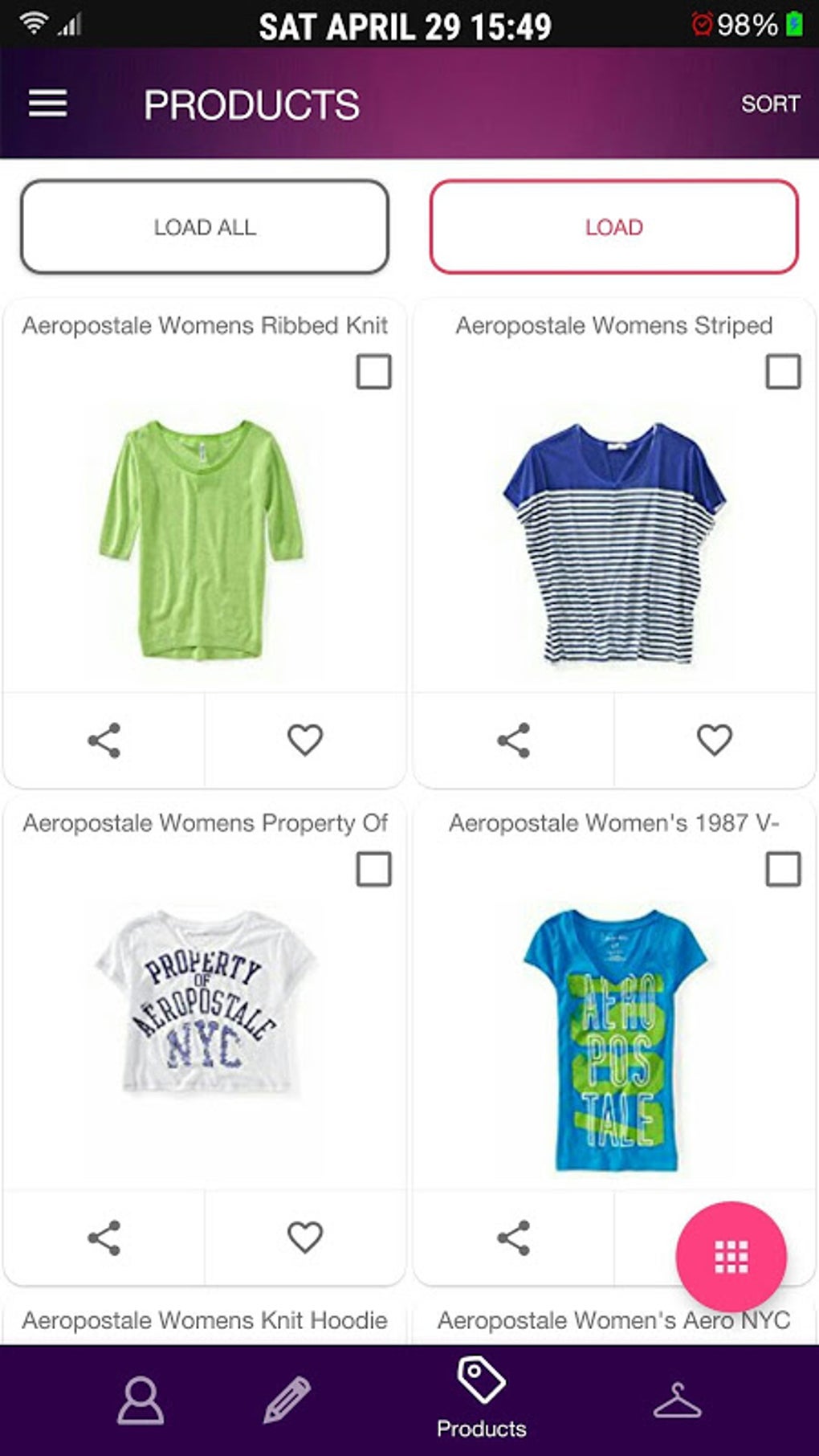Detailed screenshot of a cell phone displaying a products page. At the top of the screen, the status bar indicates it is Saturday, April 29th at 15:49, with a battery level at 98%. The Wi-Fi and reception icons are visible, signifying connectivity.

Beneath the status bar, a thin banner labeled “Products” provides a heading for the page. On the top left corner of this banner, an icon comprised of three horizontal lines, one stacked on top of the other, represents the menu.

Directly below this, a “Load All” button is positioned to the left, accompanied by a “Load” button to the right. The primary section of the page showcases the available products, arranged in a two-by-two grid.

The top left product is detailed as an Aeropostale women's ribbed knit item. Adjacent to it, on the right, is a women's striped item. The bottom row contains two more products: on the left, an Aeropostale women's "Property Of" item, and to the right, a women's 1987 V-neck shirt.